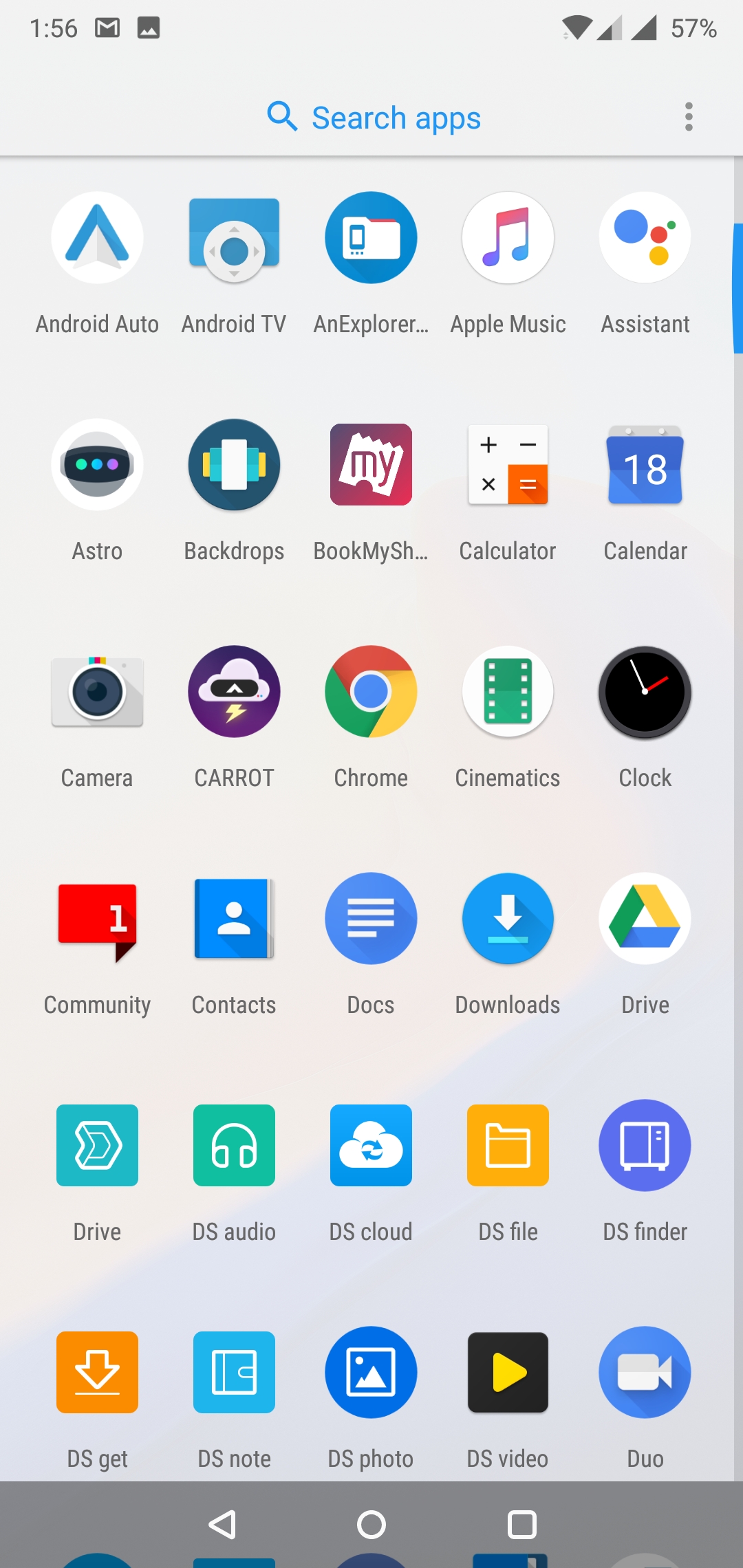The image displays the app drawer of a smartphone, featuring various application icons neatly arranged in a five-column by six-row grid. At the top of the screen, a blue "Search Apps" bar allows users to find specific applications quickly. Below is a detailed enumeration of the apps in each column:

**First Column (Left Side):**
1. **Android Auto** – Icon in white and blue.
2. **Astro** – Icon in white and gray.
3. **Camera** – Icon in gray, white, and black.
4. **Community** – Icon in red and white.
5. **Drive** – Icon in blue and white.
6. **DS Cat** – Icon in orange and white.

**Second Column:**
1. **Android TV** – Icon in blue and white.
2. **Backdrops** – Icon in blue, white, green, black, and yellow.
3. **Contacts** – Icon in blue and white.
4. **Audio** – Icon in green and white.
5. **Asstic** – Icon in blue and white (likely a mistyped or incorrect application name).

**Third Column:**
1. **Explorer** – Icon in blue and white.
2. **BookMy** – Icon in red and white.
3. **Chrome** – Icon in Google colors (blue, red, yellow, green).
4. **Docs** – Icon in blue and white.
5. **Cloud** – Icon in blue and white.
6. **Photos** – Icon in blue and white.

**Fourth Column:**
1. **Apple Music** – Icon in blue, white, and pink.
2. **Calculator** – Icon in white, black, and orange.
3. **Cinematics** – Icon in green and white.
4. **Download** – Icon in blue and white.
5. **DS File** – Icon in orange and white.
6. **DS Video** – Icon in black and orange.

**Fifth Column (Top Right):**
1. **Assistant** – Icon in Google colors.
2. **Calendar** – Icon in blue and white.
3. **Block** – Icon in black, white, and red.
4. **Drive** – Icon in blue, green, yellow, and white.
5. **DS Finder** – Icon in blue and white.
6. **Duo** – Icon in blue and white.

The overall layout provides an organized and visually balanced arrangement of frequently used applications, aiding users in easy navigation and quick access.